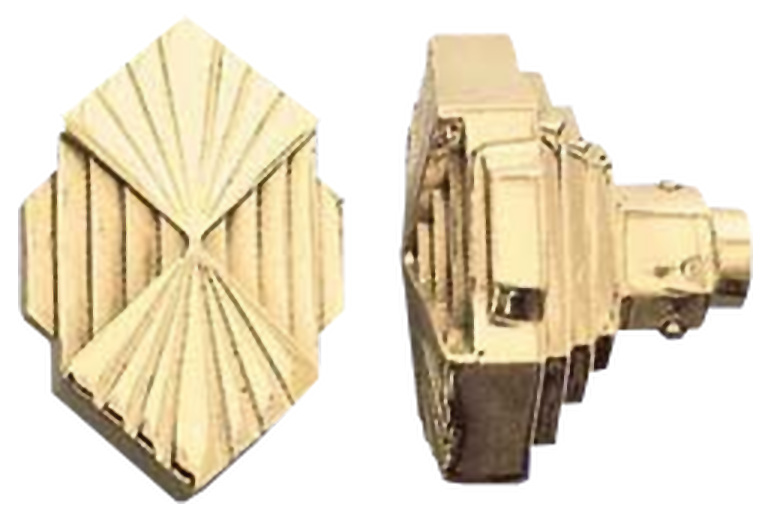The image depicts two golden decorative objects on a plain white background. The objects feature a diamond-like shape with intricate, layered detailing. The left object is shown from a top-down perspective, revealing a flat front with engraved starburst patterns and recessed stripes that resemble a stepped design, leading out to small parallelograms on the sides. This light brown, gold-colored piece shows complex texture and craftsmanship indicative of high-quality metalwork. In contrast, the right object presents a side view of the same item, unveiling its three-dimensional structure. It has pointed top and bottom ends, and its side extends outward and narrows down into a cylindrical area that appears blocky, possibly suggesting it could be plugged into another item. The precise purpose of these objects remains ambiguous, though they could potentially serve as decorative elements, caps, or covers, crafted to fit into a larger design or installation, either in a household or another setting.